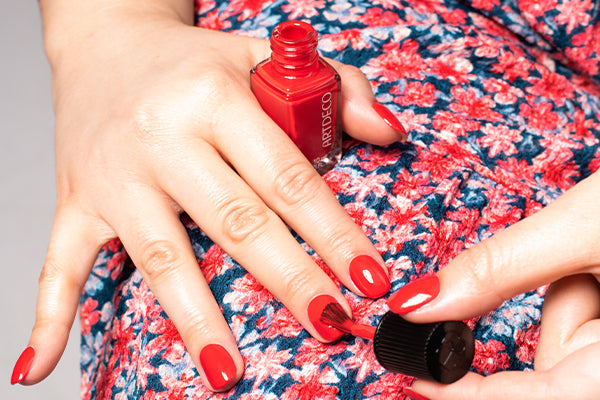This photograph is a very close-up shot of a white woman applying red, glossy fingernail polish to her nails, which are moderately long. The focus is on her hands and part of her attire. Her right hand rests on her blue skirt adorned with bright red flowers, with fingers splayed out and holding a bottle of nail polish labeled 'Art Deco' between her thumb and pointer finger. The color of the polish has a hint of orange. Her left hand, shown in part with just the thumb and forefinger visible, is holding the cap of the nail polish bottle and brushing the middle fingernail of the right hand. All the nails are already painted the same shiny red color. The image captures intricate details, emphasizing both the painting process and the floral-patterned clothing.